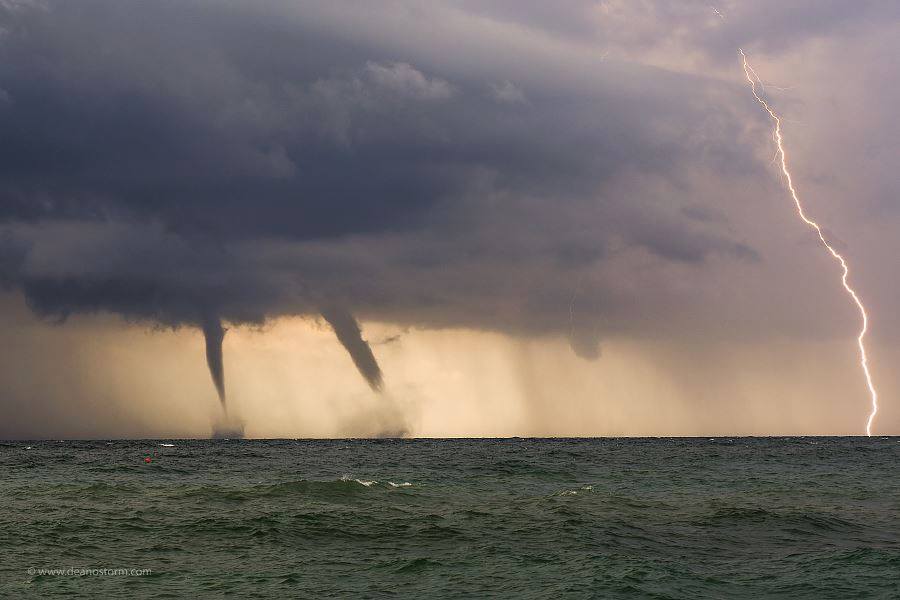This dramatic photograph, with the watermark www.deanostorm.com in the lower left corner, captures an intense storm over a tumultuous sea. The foreground showcases violent, choppy waves under a dense storm cloud. Notably, two wide water spouts, resembling full-fledged tornadoes, extend from the cloud and make contact with the ocean, causing visible updrafts of water. To the right, a third funnel cloud is beginning to form. The scene is further electrified by a lightning bolt striking the water, highlighting the storm's ferocity. No vessels are present, but some weather buoys or balloons can be seen on the water's surface, adding to the chaotic beauty of this ominous seascape.